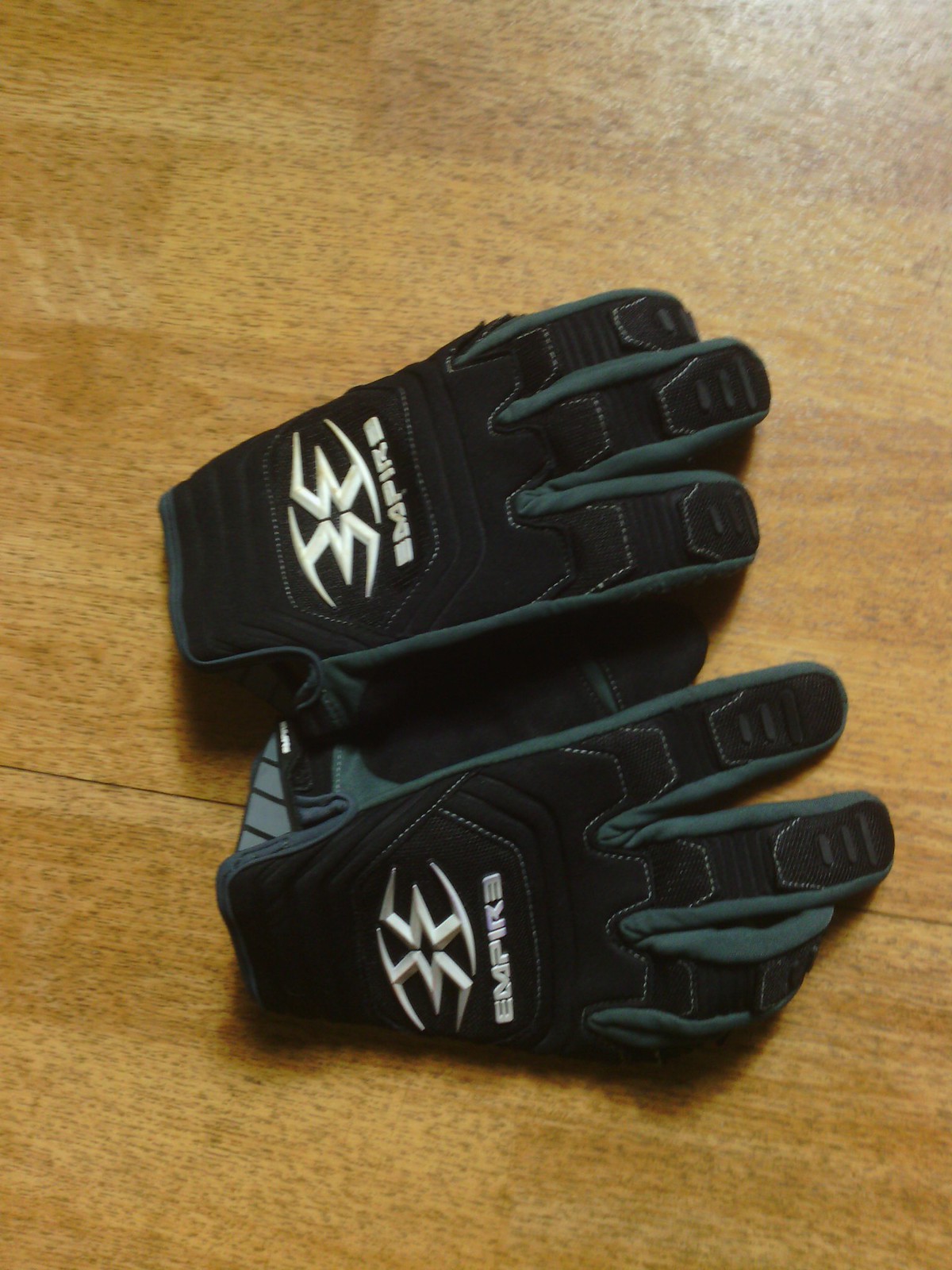This image depicts a pair of black riding gloves, which are typically used in motorsports or dirt biking. The gloves are lying flat on a medium to light-colored wooden table, arranged with their fingers pointing to the right; one glove positioned toward the top and the other toward the bottom of the picture. These gloves are characterized by their wider design with extra padding, making them suitable for high-impact activities.

The gloves feature a distinctive white design on the back, resembling two mirrored number threes connected at the center, with circles at the top and bottom. Additionally, both gloves display the word "Empire" in large white text, with the first and last 'E' stylized differently—the first 'E' is normal while the last 'E' is backwards. The gloves incorporate gray trim, particularly around the outside edges of the fingers and parts of the palms, and although they are primarily black, the contrasting gray and white elements create an eye-catching design. Interestingly, the gloves appear to have spaces for three fingers, with no visible slots for thumbs, suggesting a unique or specialized design.